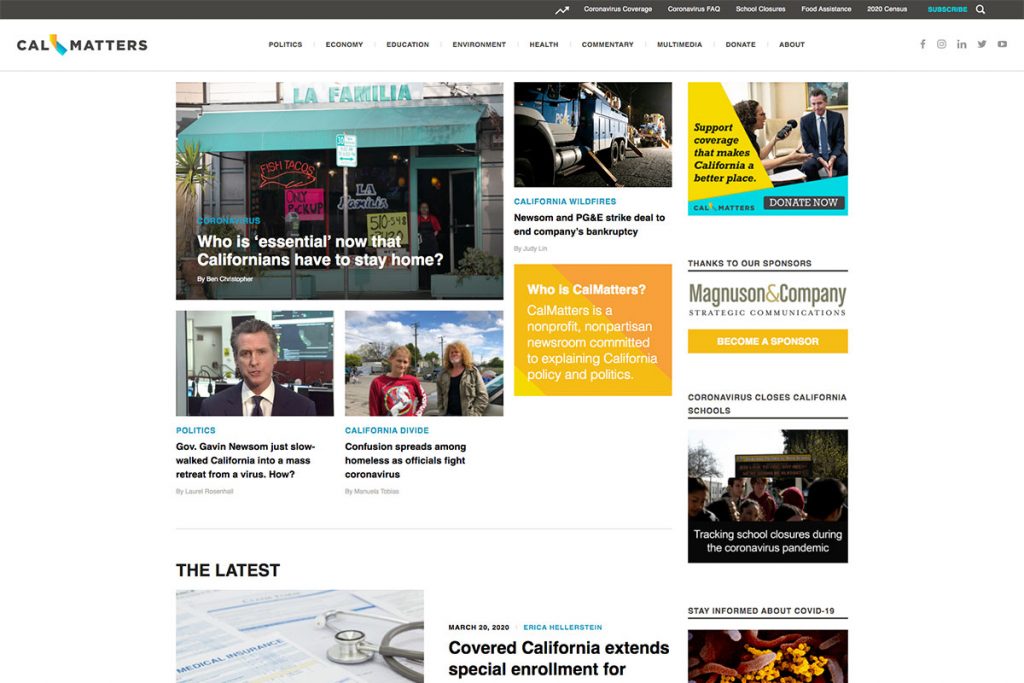The web page belongs to CalMatters, a California-focused non-profit, nonpartisan newsroom.

### Top Navigation Bar:
At the top, a black rectangular bar contains several white icons and headers. From left to right:
- A jagged line icon, resembling a mountain peak or a point.
- Headers for "Coronavirus Coverage," "Coronavirus FAQ," "School Closures," "Food Assistance," "2020 Census," and "Subscribe," with the "Subscribe" option highlighted in blue.
- A white magnifying glass icon indicating a search function.

### Logo and Main Menu:
Below the black bar is a gray rectangular section showcasing the CalMatters logo. The main menu headers are:
- Politics
- Economy
- Education
- Environment
- Health
- Commentary
- Multimedia
- Donate
- About

Social media icons for Facebook, Instagram, LinkedIn, Twitter (or X), and YouTube are located next to the main menu.

### Featured Articles:
The page displays a series of eight images with corresponding articles:
1. **La Familia:** Depicts a restaurant with the caption, "Who is essential now that Californians have to stay home?"
2. **Politics Section:** Features an image of Governor Gavin Newsom with the caption, "Governor Gavin Newsom just slow-walked California into a mass retreat from a virus. How?" The author’s name is displayed in small, gray text.
3. **California Divide:** Shows a woman and possibly a young girl, with the caption, "California divide. Confusion spreads among homeless as officials fight coronavirus."
4. **Wildfires and Politics:** Picture relating to "California wildfires, Newsom, and PG&E strike a deal to end company bankruptcy."

### Informational Box:
In the center, a vibrant yellow box in varying shades of yellow features the text:
"Who is CalMatters? CalMatters is a nonprofit, nonpartisan newsroom committed to explaining California policies and politics." This text appears in white.

### Support and Donation:
In the top-right corner, a yellow triangle with a truncated point features the message: "Support coverage that makes California a better place." A blue background with a sloped line at the bottom contains a "Donate Now" button and the CalMatters logo. Below, an image shows a reporter conversing with a man in a blue tie, accompanied by the text "Thanks to our sponsors, Magnuson and Company, Strategic Communications," followed by a "Become a Sponsor" button.

### Additional Content:
Further down, a headline reads "Coronavirus closes California schools," alongside an image of adults outside. The caption states, "Tracking school closures during the coronavirus pandemic," followed by "Stay informed about COVID-19" and images of flowers. The date "March 29th, 2020" is shown, attributing an article about extended special enrollment to Erika Hellerstein, ending abruptly.

### Latest Updates:
A section titled "The Latest" includes an image of a stethoscope and medical insurance forms indicating recently updated content.

This detailed breakdown captures the structural and thematic elements of the CalMatters homepage, reflecting its focus on California news and public interests.